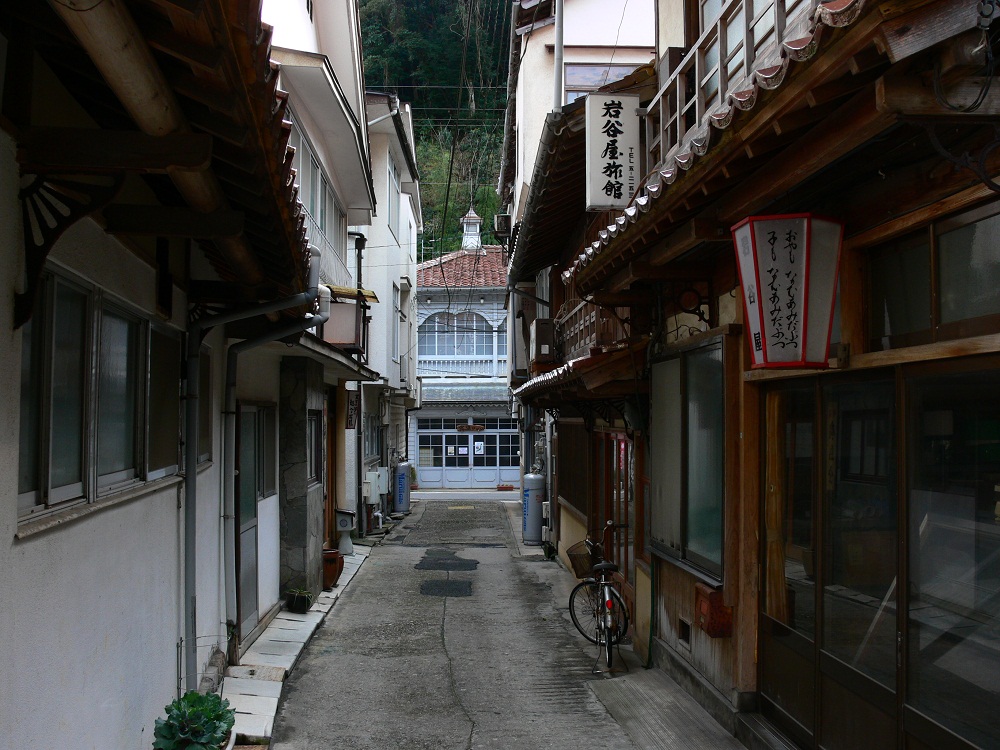The image depicts a dimly lit, narrow alleyway, potentially located in an Asian city based on the presence of kanji characters on the signs. The alleyway is paved with cracked cement and flanked by a series of continuous buildings on both sides, illustrating traditional Asian architectural elements such as wooden walls, tiled roofs, and distinctive windows. On the left side, there are multiple stories of dwellings, including a visible two-story building and narrow doors with plants by the entryways. The right side features shop windows adorned with Asian script, lanterns, and a bicycle with a brown basket parked in front. Moving towards the end of the alley, a prominent two-story building with a balcony and a clay-tiled roof comes into view, complemented by a cupola. Further beyond this building, tall green trees create the impression of a forested hillside. Additional details include a propane or gas tank near the end of the alley and the general ambiance of an intimate urban passageway.